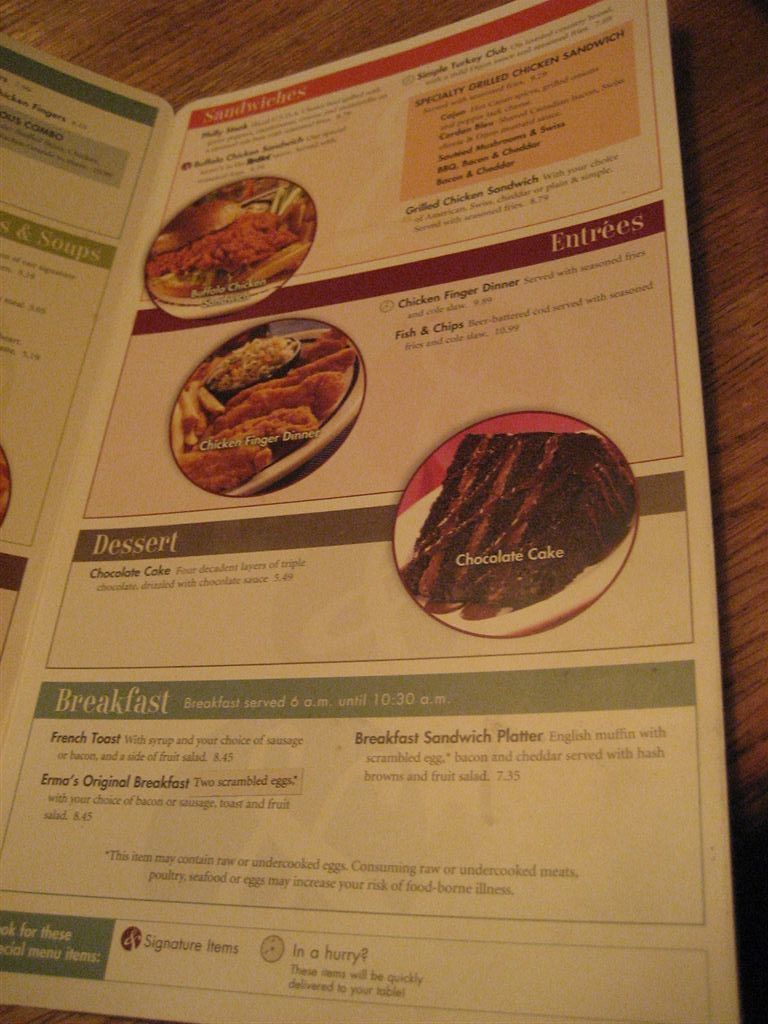A rustic brown wooden table at a dimly-lit restaurant holds a detailed menu. This menu is divided into several sections: breakfast, entrees, desserts, sandwiches, and soups. Breakfast is served from 6:00 to 10:30 AM, offering three different options. The dessert menu lists a single item—decadent chocolate cake. For entrees, diners have two meat-centric choices: chicken finger dinner or fish and chips. The sandwich section boasts four varieties, including specialty chicken sandwiches like Cajun and Cordon Bleu, BBQ bacon and cheddar, and a simple bacon and cheddar option.

The menu is visually rich, featuring images of some highlighted dishes: a tempting buffalo chicken sandwich, crispy chicken fingers, and the luscious chocolate cake. However, the breakfast items have no accompanying images. The warm ambiance and thoughtfully laid-out menu promise a comforting dining experience.